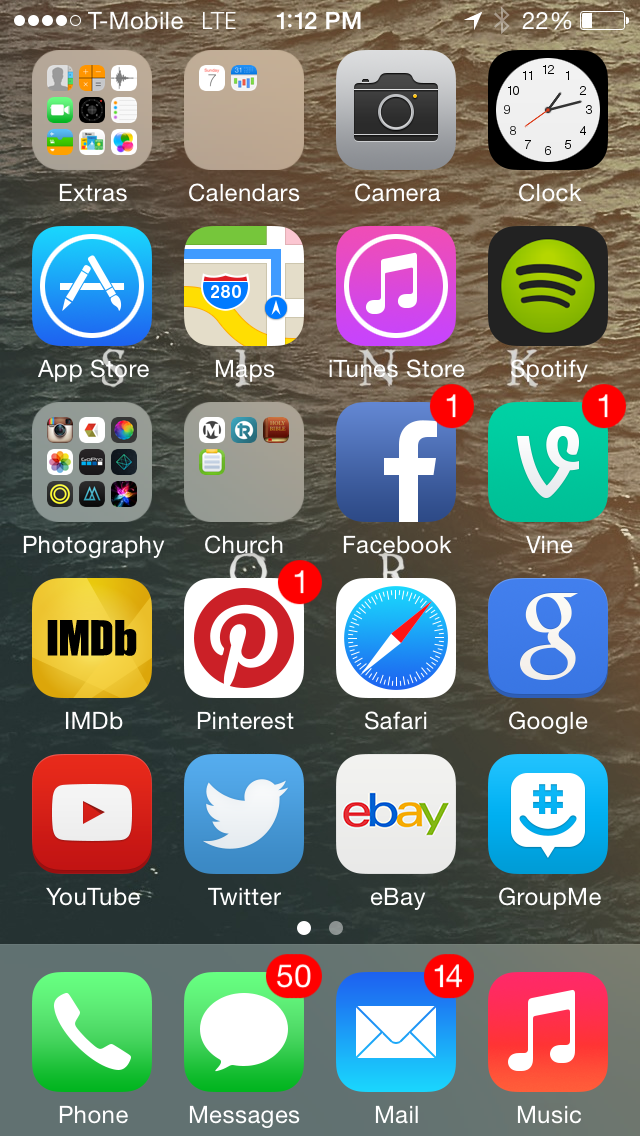Here is a detailed and cleaned-up caption for the image:

---

The image displays a smartphone screen with various elements and app icons. At the top of the screen, the status bar shows four solid white circles and one hollow circle, indicating the cellular signal strength. To the right, it displays "T-Mobile LTE," the time "1:12 PM," and the battery level at 22%. The home screen is organized into five rows, each containing four app icons. From top to bottom, the first row includes "Extras," "Calendar," "Camera," and "Clock." The second row features "App Store," "Maps," "iTunes Store," and "Spotify." The third row displays "Photos," "Church," "Facebook," and "Vine," with Facebook, Vine, and Pinterest showing red notification circles with white numbers indicating unread notifications. The fourth row consists of "IMDb," "Pinterest," "Safari," and "Google," while the fifth row includes "YouTube," "Twitter," "eBay," and "GroupMe." Each app is represented by its respective icon. 

At the very bottom of the screen, the fixed dock contains four primary apps: "Phone," "Messages," "Mail," and "Music." The "Messages" app icon shows 50 unread messages, and the "Mail" app icon shows 14 unread emails. The background image is a close-up of a rippling water surface with a brownish hue, providing a serene backdrop to the app icons.

---

This comprehensive caption includes the specifics of the screen layout and all the relevant details mentioned.